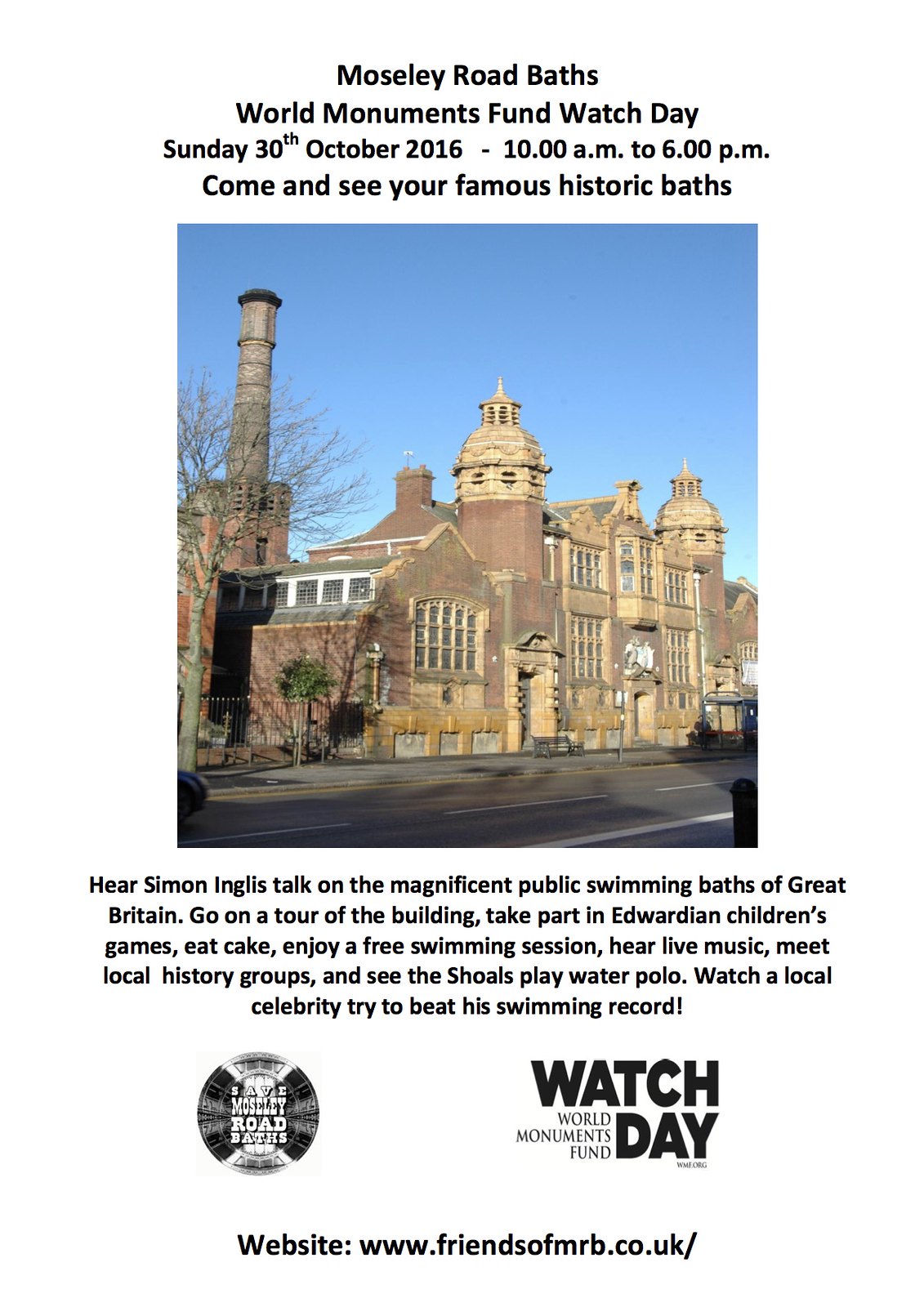The image depicts a historic brick building under a clear blue sky in an old city, captured from a distance. The building, characterized by various shades of brown and gold and numerous windows, is identified as Moseley Road Baths in England. The scene includes the building with a backdrop of trees. Above the photograph, text in black on a white background announces "Moseley Road Baths, World Monuments Fund Watch Day, Sunday 30th October 2016, 10 a.m. to 6 p.m. Come and see your famous historic baths." Below the image, additional text invites people to hear Simon Inglis discuss the magnificent public swimming baths of Great Britain, join a tour of the building, participate in Edwardian children's games, eat cake, enjoy a free swimming session, hear live music, engage with local history groups, watch the Shoals play water polo, and see a local celebrity attempt to beat his swimming record. At the bottom of the advertisement are two logos: one for "Save Moseley Road Baths" and another for "Watch Day, World Monuments Fund." The website www.friendsofmrb.co.uk is also prominently displayed.